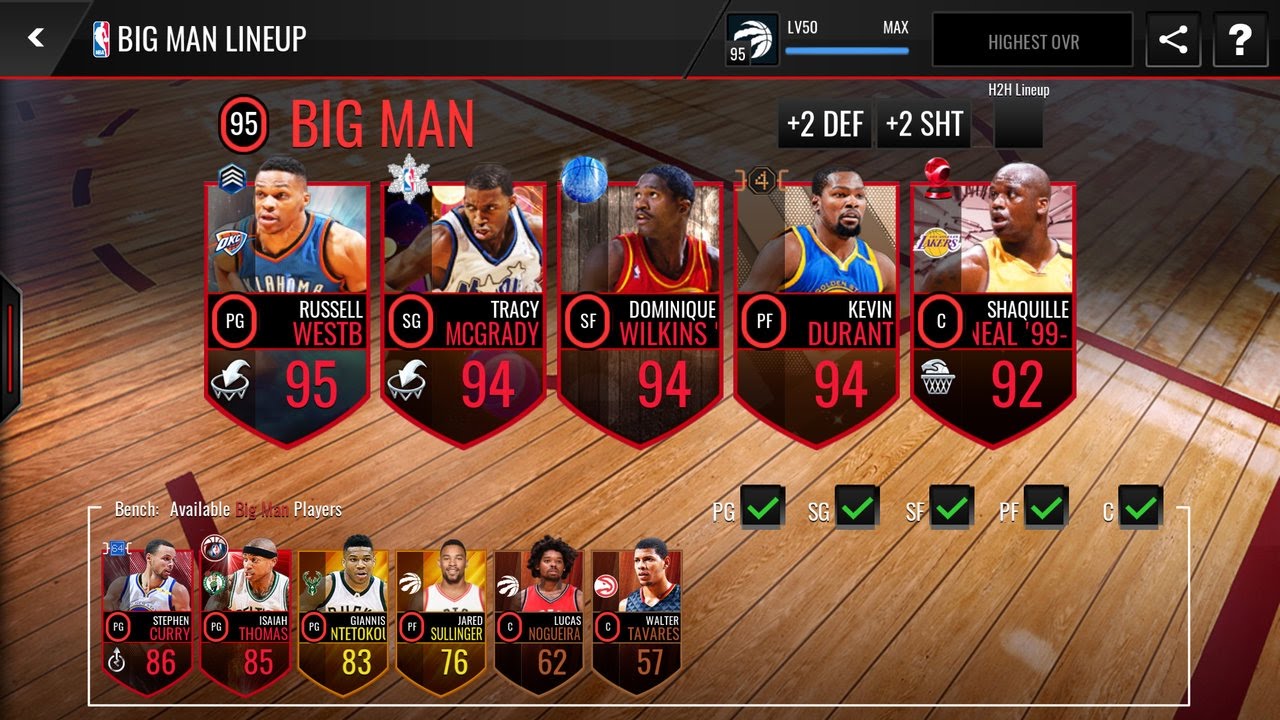This image is from the "Big Man" lineup series. At the upper left-hand corner, the title "Big Man lineup" is prominently displayed, accompanied by an NBA logo to its immediate left and a back arrow further to the left, indicating navigation options. The theme of the image is basketball, reflected in the background which depicts a close-up view of a basketball court with a slightly dark ambiance highlighting the wooden floor.

At the top of the image, a semi-transparent black bar spans across, where on the far right, the level is indicated as 50, which appears to be the maximum level, complemented by a blue progress bar beneath it. Adjacent to this, there's a block displaying the highest OVR (Overall Rating), alongside a share button and a help/question button.

The main focal point of the image showcases the lineup of five basketball players: Russell Westbrook, Tracy McGrady, Dominique Wilkins, Kevin Durant, and Shaquille O'Neal. Each player is positioned prominently, celebrating their inclusion in this elite lineup.